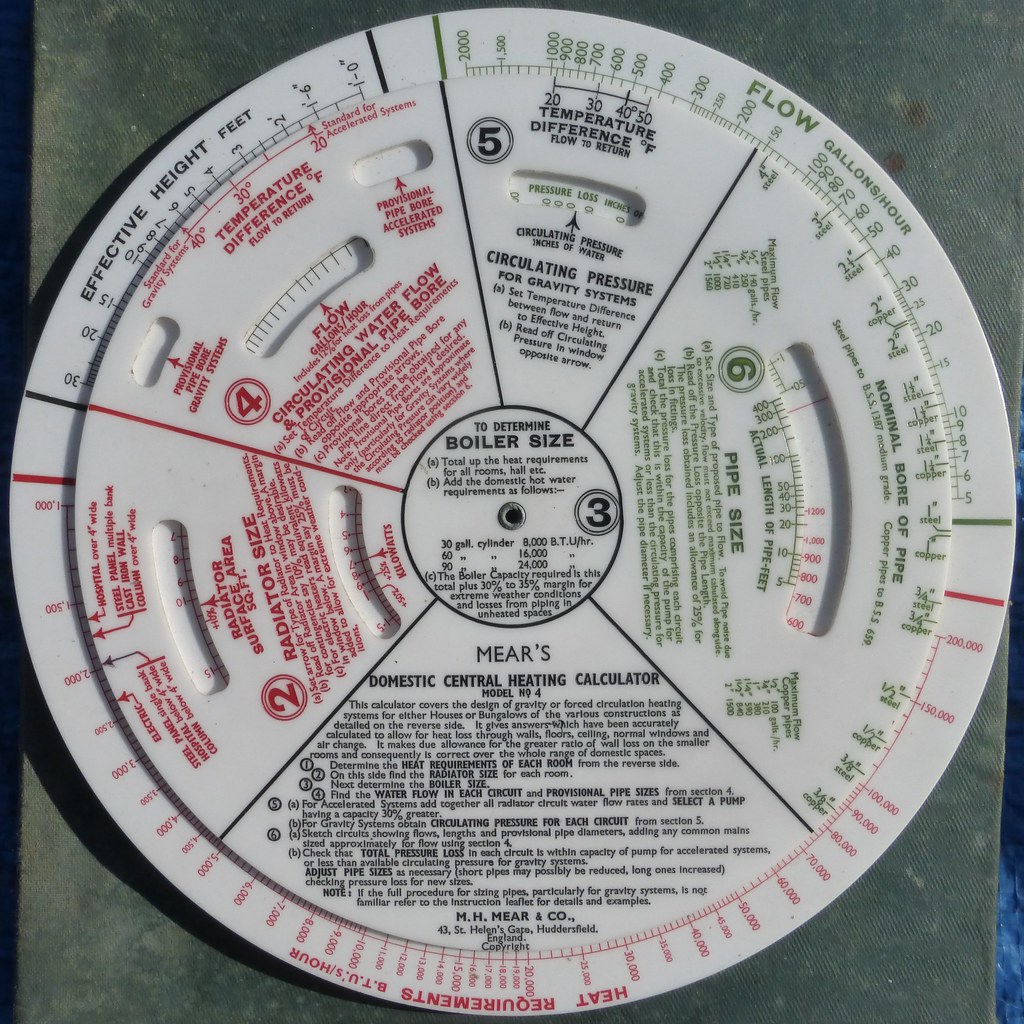The image depicts a highly detailed, plastic measuring device centered on a concrete background. The device is a circular dial, resembling a pie chart with multiple colored sections and detailed instructions. It is used to determine the appropriate boiler size for various heating requirements. The outer circle features multiple numbers in different colors—green for flow (measured in gallons per hour), red for heat requirements (measured in BTUs per hour), and black for effective height (measured in feet). The dial is segmented into quadrants like a clock face, with each quadrant providing specific data and instructions. In the center, there is a larger circular section that provides the critical instruction: "to determine boiler size, total up the heat requirements for all rooms, add the domestic hot water requirements." The inner circle is rotatable, overlaying the outer circle with cutouts and additional numeric details. This device is likely used by technicians to calculate the needed boiler size for various domestic applications, such as heating systems in buildings like hotels or residential homes. A metal clip at the center indicates that the dial can be rotated to align different values for accurate measurement.